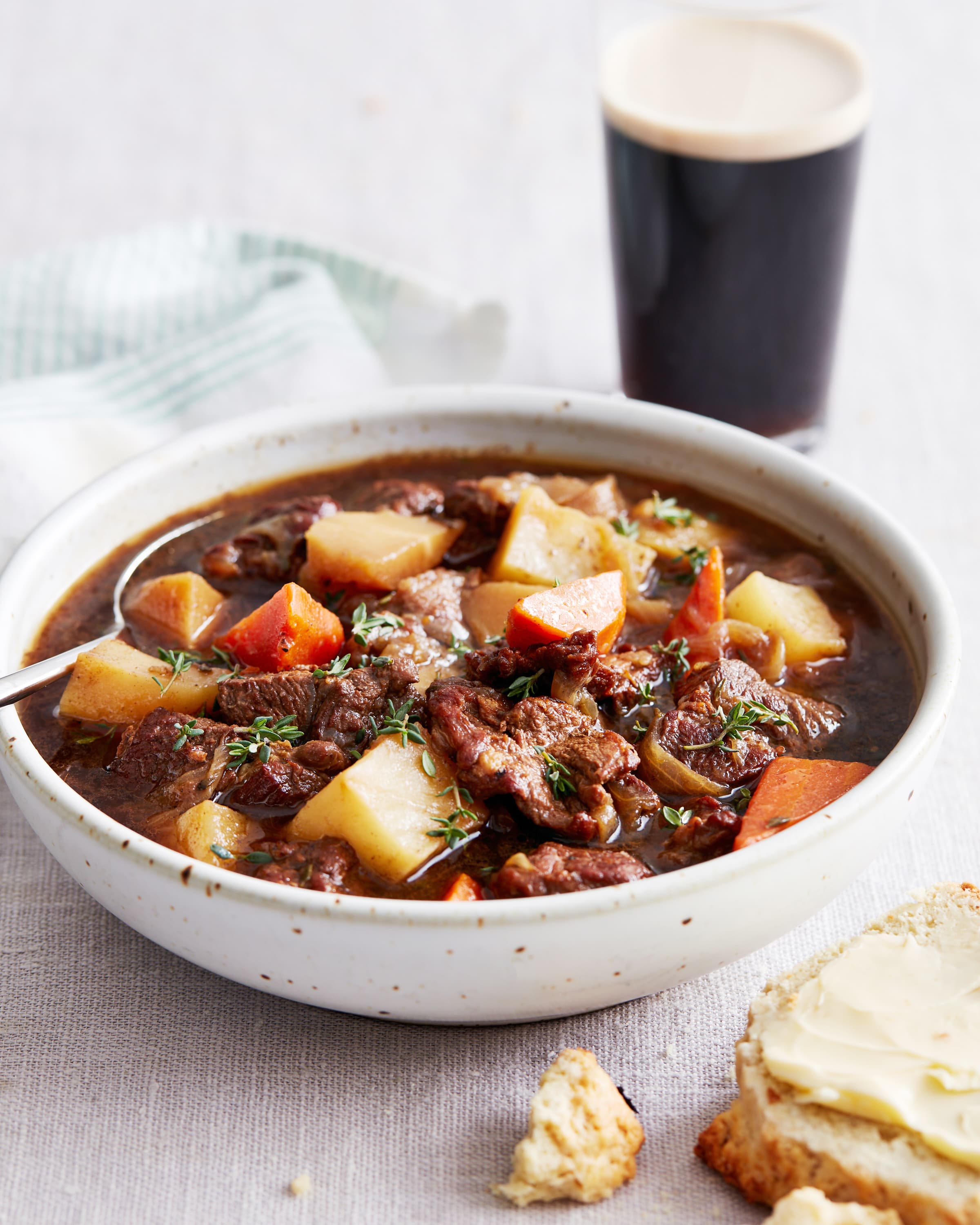The image captures a hearty Irish stew presented in a deep white bowl adorned with brown specks. The stew consists of large chunks of beef, potatoes, and carrots, all immersed in a thick, dark brown broth. Fresh green herbs are lightly sprinkled on top, enhancing its rustic appearance. To the bottom right of the bowl, there is a piece of bread generously smeared with butter, with a smaller piece torn off and placed to the left. The bowl is situated on a linen tablecloth, and a spoon is inserted into the stew. In the background, slightly blurred due to depth of field, stands a tall glass filled with a dark beverage topped with a frothy head, possibly a pint of Guinness. Adjacent to the drink, to the left, is a blue- and white-striped fabric napkin. The photo is taken at an angle, providing a comprehensive view of the inviting meal and its surroundings.